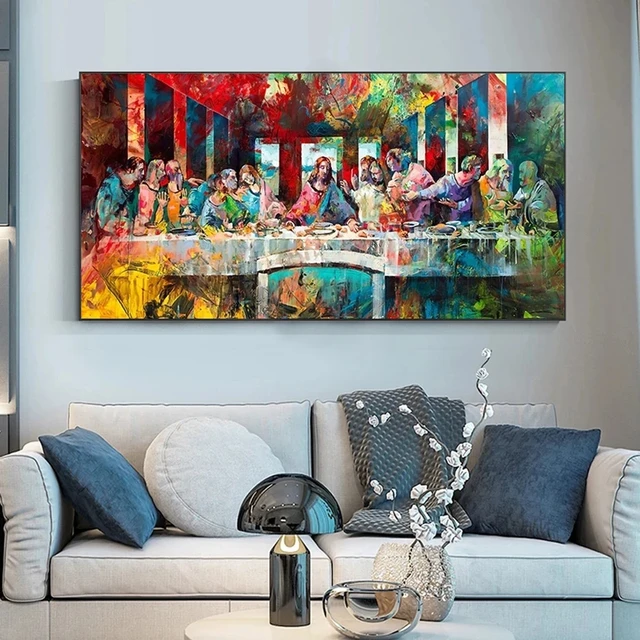The photograph captures a meticulously decorated living room with a contemporary, light gray upholstered two-cushion sofa adorned with darker gray accent pillows on each side and a round gray pillow in the center. A dark gray throw blanket is folded and draped over the back of the sofa. In front of the sofa is a round, white coffee table that holds a shiny, black dome-shaped lamp reflecting the room's details, a clear glass bowl, and a vase filled with ornate long twigs and white flowers. The backdrop to this setting is a white painted wall featuring an expansive, rectangular acrylic painting of the Last Supper. The vibrant and abstract rendition of Jesus and the disciples is accented with splashes of reds, yellows, greens, and blues, creating a visually stunning and modern piece that spans the length of the sofa. This contemporary and modern stylized room exudes elegance and tasteful design.